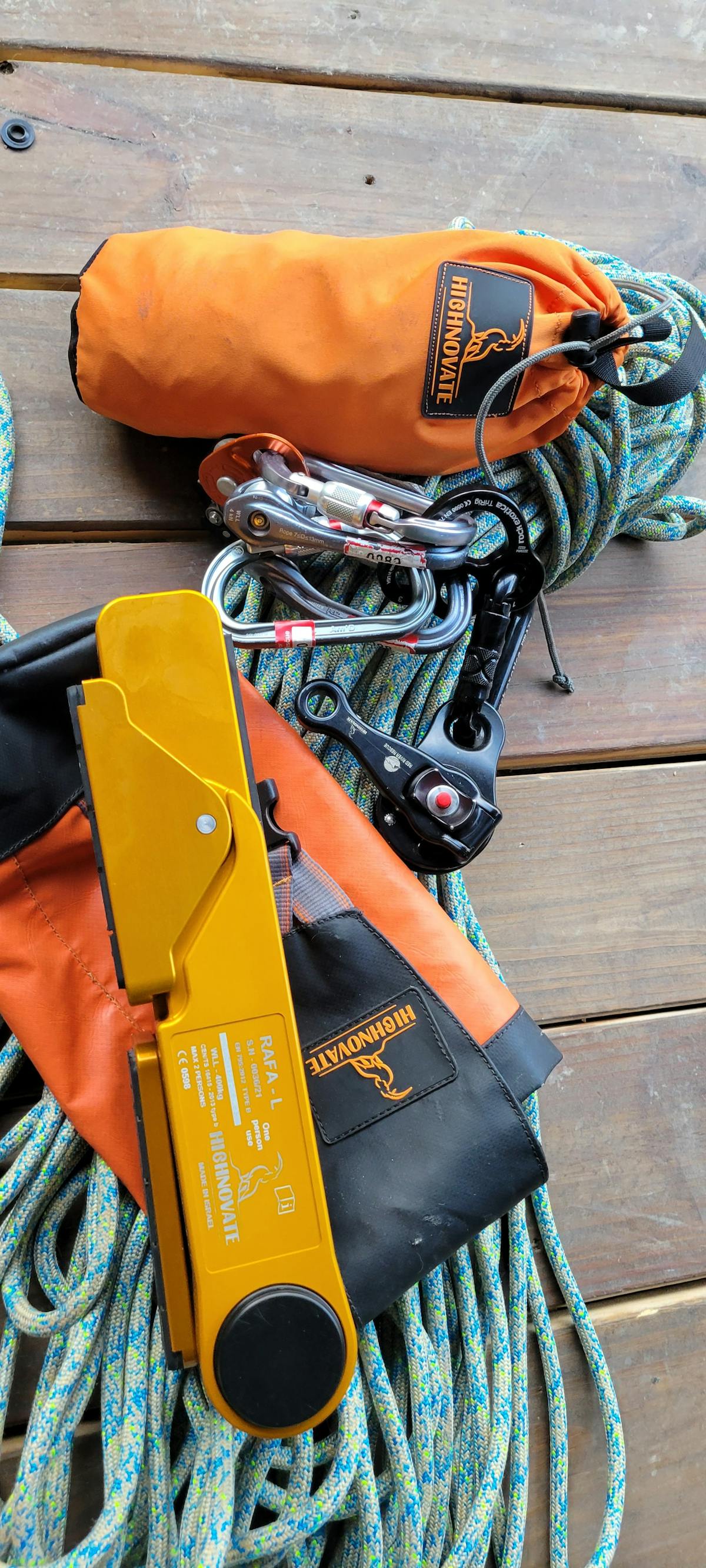The image depicts a collection of rock climbing or bungee jumping gear laid out on a dark brown wooden deck or pier. Dominating the scene are two orange pouches, both emblazoned with the brand name "Hi Novete." The equipment includes thick, multicolored ropes featuring shades of blue, green, gray, and white, wound together in a bundle. Also visible are various types of carabiners and clips, some adorned with red stickers, likely for safety harnesses. Among the gear is a yellow device of uncertain purpose. The Hi Novete brand is prominently displayed both on the orange pouches and on some of the clips, adding a cohesive element to the assortment of cables and tools.